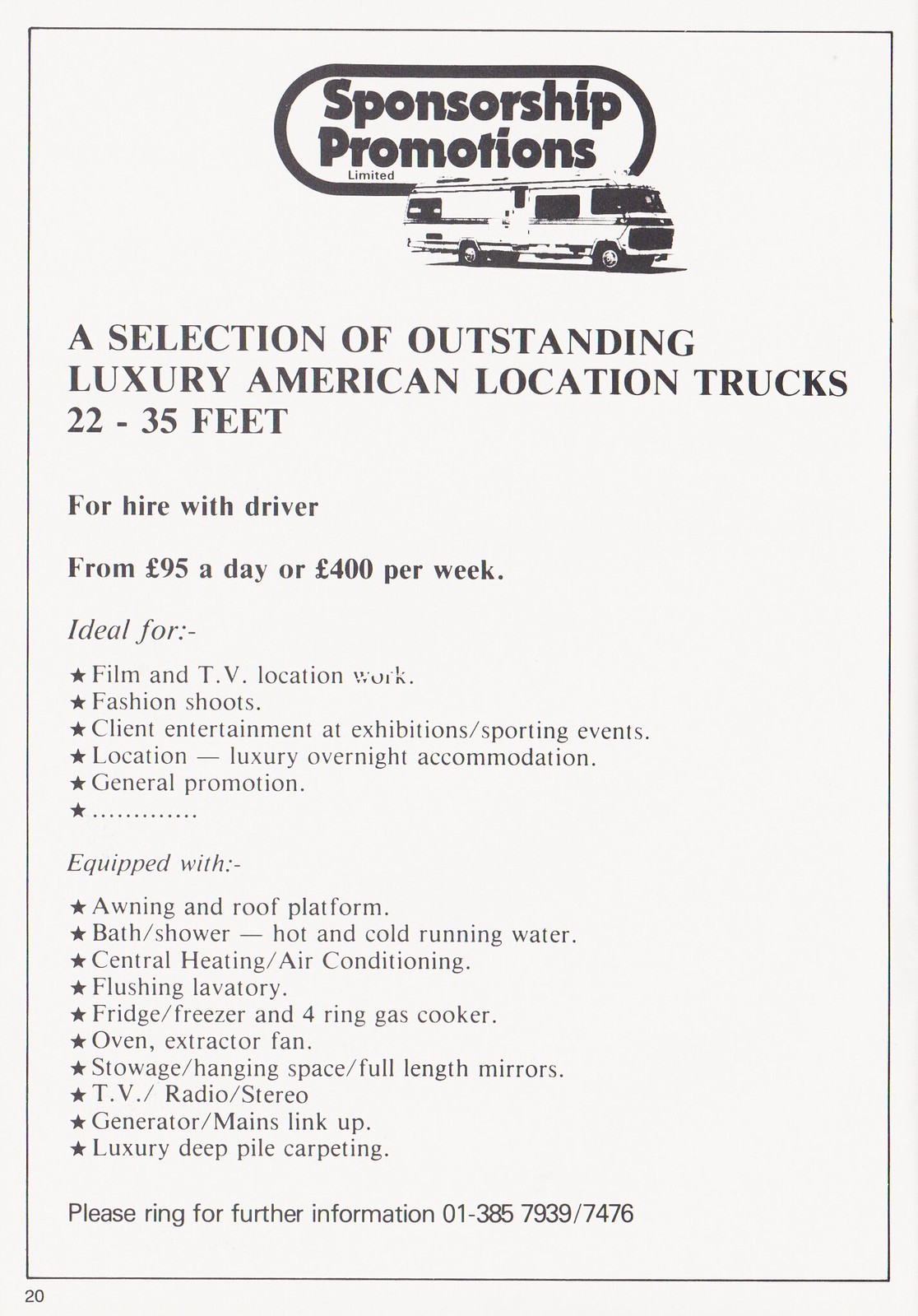The advertisement features a white background adorned with black text and images. At the top, "Sponsorship Promotions Limited" is prominently displayed alongside a picture of a luxury RV, or Winnebago. The text below highlights a selection of outstanding luxury American location trucks available for hire, ranging from 22 to 35 feet in length, with a driver provided. Prices are quoted at £95 per day or £400 per week. The RVs are pitched as ideal for film and TV location work, fashion shoots, client entertainment, exhibitions, and sporting events. The vehicles are described as being equipped with a range of amenities, including an awning and roof platform, bath/shower, hot and cold running water, central heating and air conditioning, flushing lavatory, fridge/freezer, four-ring gas cooker, oven, extractor fan, stowage, hanging space, full-length mirrors, TV, radio, stereo, generator, mains link-up, and luxury deep pile carpeting. For further information, readers are encouraged to call 01-385-7939-7476. The page is likely from a pamphlet or magazine, and the layout includes multiple ellipses and stars as bullet points.